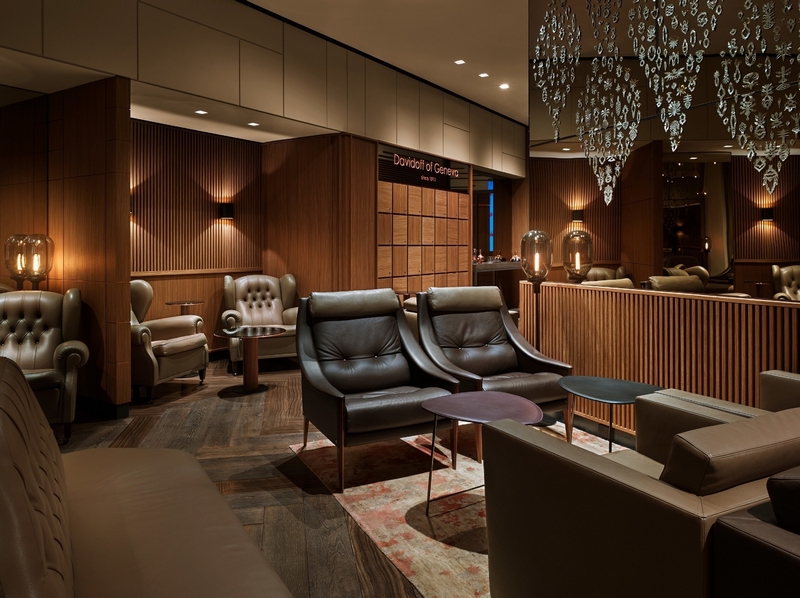This photograph captures the opulent interior of what appears to be an exclusive, high-end lounge or perhaps a gentlemen's club named "Davidoff of Geneva," as indicated by the sign posted on the wall in the background. The room is lavishly styled with rich, warm brown tones consisting primarily of wood-paneled walls and dark leather furniture, creating a masculine and sophisticated ambiance. The seating arrangement in the mid-ground features several leather chairs in varying shades of brown and gray, accompanied by small coffee tables. These chairs are meticulously placed with two dark brown leather chairs on one side and two lighter brown chairs on the opposite side. The left wall features cubby-like structures. The flooring is made of wood, adding to the overall warmth of the space. Sconces and large filament light bulbs scattered throughout the room cast a cozy, inviting glow, enhancing the space's intimacy. A decorative etched glass on the window or mirror to the right adds a subtle touch of elegance. The ceiling lights resemble high-end fixtures, possibly chandeliers, further emphasizing the luxurious atmosphere of this exquisitely decorated establishment.